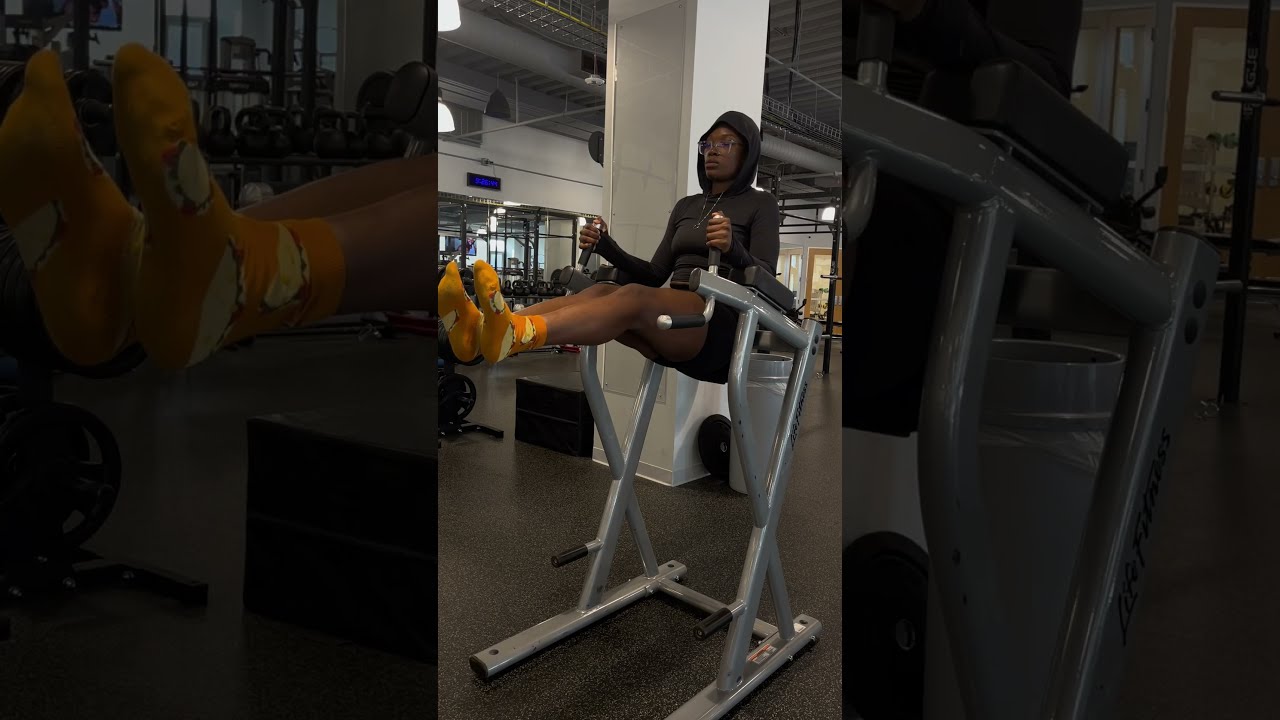In a spacious gym with an industrial, unfinished ceiling revealing pipes and scaffolding, an African-American woman is captured mid-exercise on a sleek, gray pull-up machine designed for ab workouts. She holds a raised, seated position with her legs extended straight out in front of her, supported by her arms resting on the armrests and gripping the vertical handles. Her attire consists of black exercise shorts and a form-fitting, long-sleeved black hoodie, with the hood pulled up over her head. She also sports glasses, a gold chain, and vibrant orange socks adorned with yellow characters. Behind her is a large white column with a mirror, a gray trash can, and the rest of the gym, featuring dark gray concrete flooring and various pieces of exercise equipment. The background includes windows and a glass entryway, adding to the expansive feel of the space.